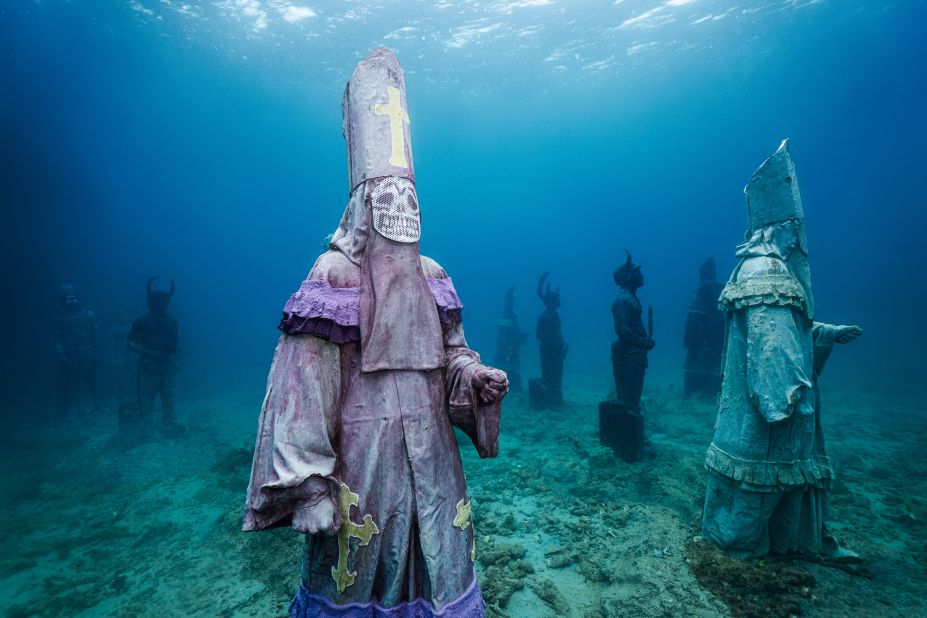The image shows a haunting underwater scene featuring several statues resembling religious figures amidst an otherworldly aquatic environment. The central statue is a man dressed in a light purple, flared suit that extends to his wrists. One of his hands hangs down to his knees, while the other is raised to his chest. His face is obscured by a white mask with black eyebrows, eyes, and an open mouth displaying teeth, topped by a gray hat with a yellow cross. To the right stands a similar statue, though colored teal, facing slightly to the right. Behind these prominent figures, a multitude of demon-like statues with devil horns can be seen, contributing to the eerie ambiance. The ocean floor is strewn with debris and seaweed, and the light from the surface filters through the water, illuminating the scene with a ghostly glow in the light blue background.